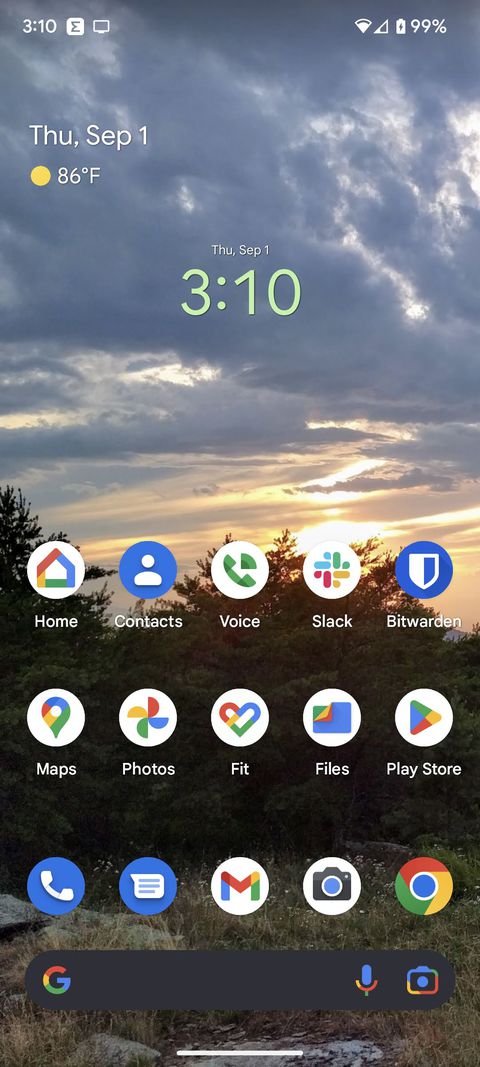This screenshot captures the homepage of a Google phone, prominently featuring Google apps. At the top left, the time is displayed as 3:10, while the top right shows status indicators for Wi-Fi, cellular signal, and battery life at 99%. Just below the clock on the left, the date reads "Thursday, September 1st" alongside a yellow sun icon and a temperature of 86°F. Centralized beneath, the date "Thursday, September 1st" is repeated alongside another clock displaying 3:10.

The wallpaper showcases a picturesque sunset with a cloudy sky above a landscape of grass and bushes. The app icons arranged on the screen include Google Home, Contacts, Voice, Slack, Bitwarden, Google Maps, Google Photos, Google Fit, Google Files, and Google Play Store. Additionally, there are icons for Phone, Text, another Google app with an 'M' symbol, Camera, and Google Chrome.

At the bottom of the screen, a search bar with the Google 'G' logo on the left and microphone and camera icons on the right is prominently placed. Below the search bar, a white swipe-up line is visible, indicating the gesture to open or switch pages.

This detailed depiction highlights the essential elements and layout of the phone's homepage, providing a clear understanding of its interface and functionalities.